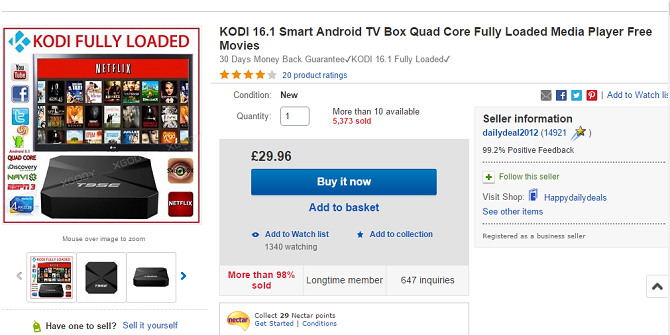**Image Caption:**

A detailed view of an online store listing for the Kodi TV box. In the top left corner, the page displays the text "Kodi Fully Loaded" in red against a bright background, highlighted by a red outlined square. Inside this section, there is an image of a TV showing the Netflix home screen featuring various movie thumbnails. Adjacent to this, social media icons for YouTube, Facebook, and Twitter are visible along with the "SPN3" and "Navi" channels.

The device for sale is a black Kodi TV box, prominently displayed with an "X Kodi" watermark. To the right, detailed product information reads: "Kodi 16.1 Smart TV Box, Quad Core, Fully Loaded Media Player, Free Movies, Day-to-Day Money Back Guarantee." The product has a rating of four stars and is listed as new with a quantity of one, more than ten available, and a total of 73 units sold out of 5000 in stock. This information is highlighted in red text.

Below this section, a blue "Buy It Now" button is shown with a price of 29.96 Euros. There are additional options including "Add to Basket," "Add to Watch List," and "Getting 40 Watching." The listing mentions that more than 98% of the items are sold by this long-time member with 647 inquiries to date.

On the right side, the seller's information is listed: "Seller Information: Daily Deal 2012-14, 9 to 1, 99.2% Positive Feedback." Options to "Follow this Seller," "Visit Shop," and "See Other Items" are also provided. This section features social media icons for email, Facebook, Twitter, and Pinterest. Lastly, the bottom left corner encourages users to "Have One to Sell? Sell it Yourself".

The text within the image is color-coded with some in blue, black, and red to emphasize various details.